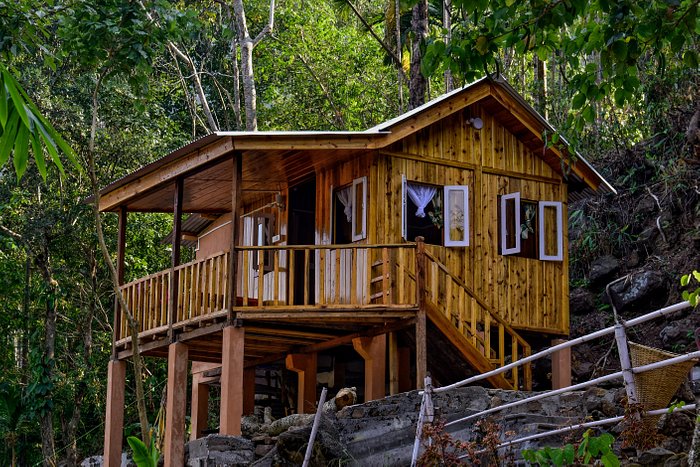The photograph depicts a quaint, one-story cabin nestled in a wooded area, likely constructed from pine or redwood, finished with a sealant such as linseed oil that gives it a noticeable sheen. The cabin is built on sturdy wooden stilts atop natural stone, preserving the surrounding landscape. It features a corrugated metal roof with an overhanging veranda, supported by large wooden pylons, creating a charming, raised porch accessible by a set of stairs. The cabin's exterior is adorned with white-accented shutters framing four visible windows, enhancing the warm, rich wood tones. Surrounded by lush, summer foliage and possibly aspen trees, this secluded retreat is encircled by a large fence, creating a serene and inviting atmosphere, perfect for a peaceful getaway.